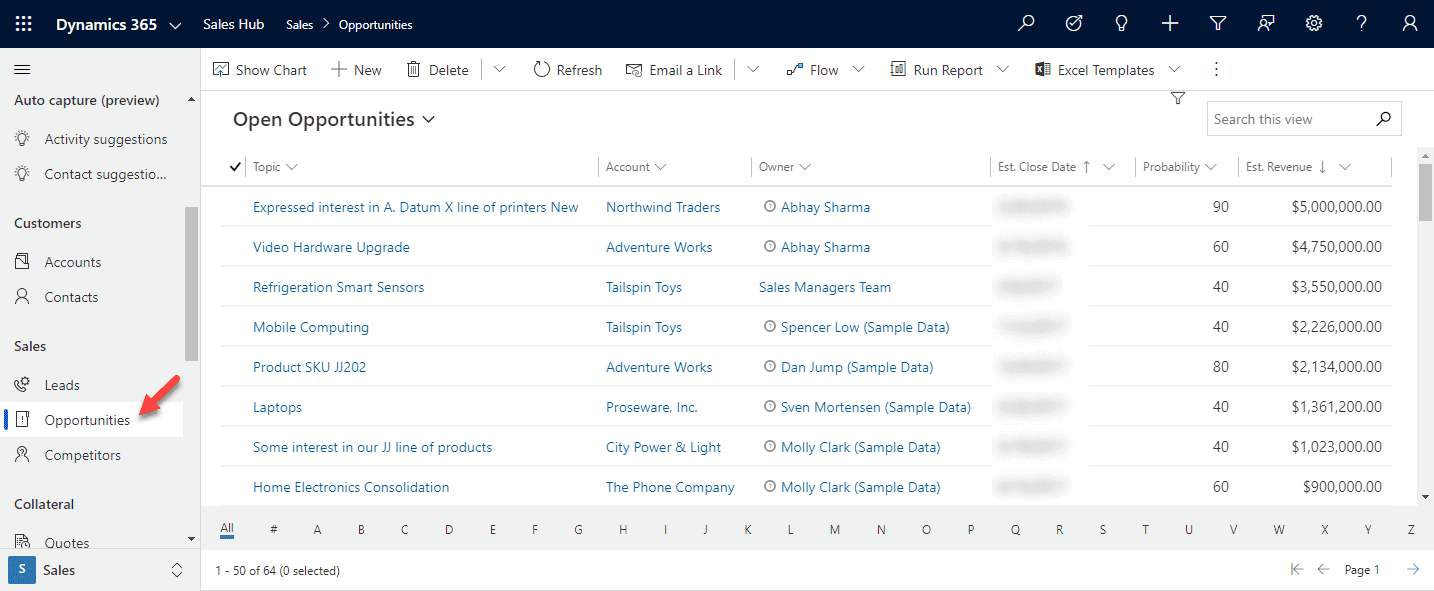The image features a detailed view of a webpage interface from Dynamics 365. The header of the webpage is dark blue and includes a menu icon along with various tabs such as Dynamic 365, Sales Hub, Sales, Opportunities. Icons for Search, Check, Ideas, Add, Filter, Settings, Help, and Profile are aligned at the top.

On the left side of the interface, there is a menu with several options: Auto Capture Preview, Activity Suggestion, Conduct Suggestion, Custom Account, Conduct, Sales, Lead, Opportunities, Competitors, Collateral, Quotes, and Sales, arranged vertically. 'Opportunities' is specifically highlighted, indicated by a blue line to its left and a red arrow pointing at it. The background of this menu is grey.

The main section of the page displays the 'Opportunities' tab which is currently open. At the top of this section, there are action tabs such as Shortcut, Glass New, Delete, Refresh, Email Link, Flow, Run Report, and Excel Template. Below this, the title 'Open Opportunities' is displayed, followed by a table that outlines various opportunities.

The table lists columns labeled: Topic, Account Owner, Estimation, Close Date, Probability, Estimated Revenue, and Revenue. The 'Topic' column includes various entries like Express Interest in a Data Mixed Line of Printers, New, Video Hardware Upgrade, Geo-Futuristic Smart Sensors, Mobile Computing, Product SKU, Laptop, Some Interest in our JJ Line of Products, Home Electronics, and Consolation. The Topic names and Account Owners are written in blue, whereas the Probability and Estimated Revenue details are in black.

This organized layout facilitates easy navigation and management of sales opportunities within Dynamics 365.